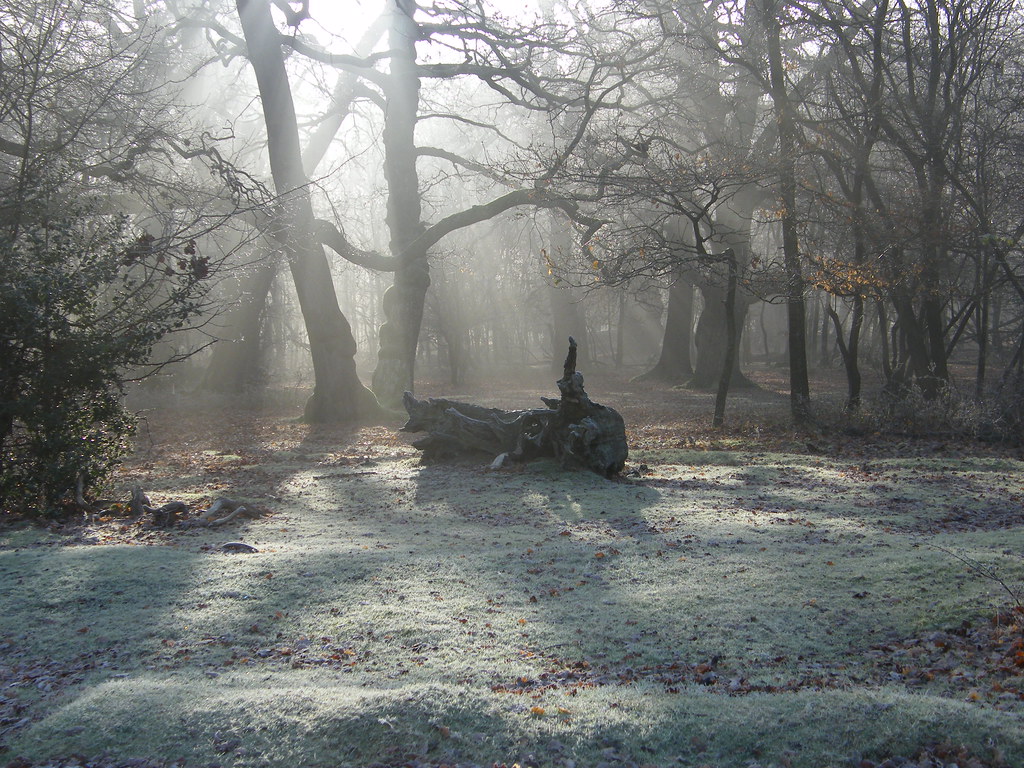This color photograph captures a serene, early morning winter scene in a wooded area. Sunlight streams through the tall, leafless trees and diffuses through a thick fog, creating a hazy, almost ethereal atmosphere. The forest floor is covered in a layer of white frost, interspersed with dead leaves. In the center of the image lies an old, burnt tree trunk, stark and solitary, lending an air of ruggedness to the tranquil surroundings. The subdued tones of brown and off-white dominate the color palette, highlighting the stark beauty of the winter landscape. The interplay of light and fog adds a touch of lightness to the otherwise stark scenery, making it a captivating and beautifully balanced photograph.